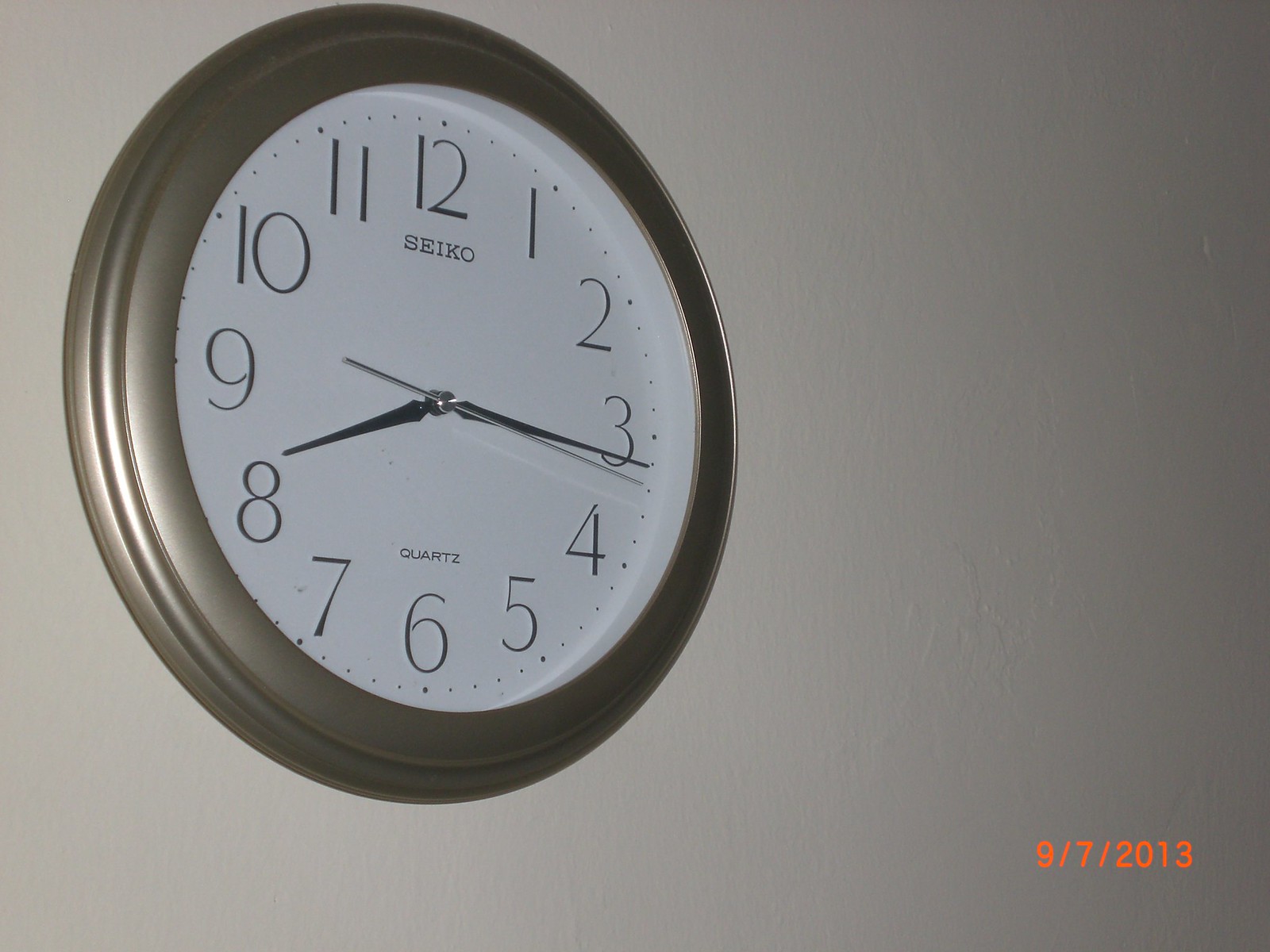This photograph captures a wall clock prominently displayed against a plain gray, drywall surface. The clock features a sleek silver frame surrounding a clean white face. Traditional numerals, starting with 12 at the top, mark each hour, with small dots serving as indicators between the numbers. The timepiece is branded "Seiko," with the logo positioned just below the 12 o'clock marker. The clock's hands—comprising the hour, minute, and second hands—are a striking shiny black, offering a sharp contrast to the white face. In the bottom right corner of the image, a date stamp reads "9-7-2013," subtly indicating the time at which the photo was taken.